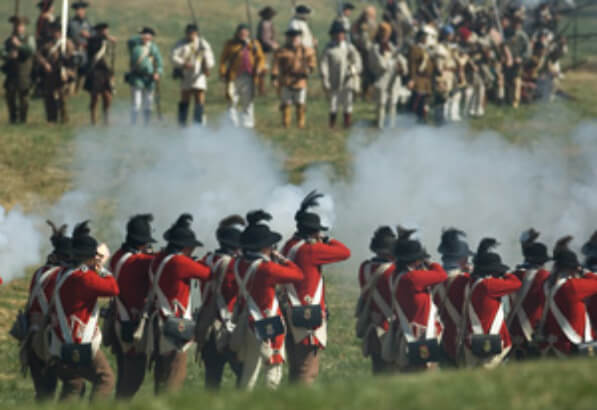The image captures a slightly blurred Revolutionary War reenactment, showcasing a scene of historical battle on a large grassy field. In the foreground, a line of soldiers dressed as British redcoats fires their muskets, producing clouds of white smoke and visible orange flashes from the gunfire. These redcoats wear distinctive red outercoats with white "X" straps across their backs, used to hold gunpowder and other military equipment. They sport black hats adorned with black feathers and are clad in a mix of white and brown pants. Accompanying each soldier is a small black bag with a gold medallion, strapped across their shoulders.

Further in the distance, another group of soldiers, representing American revolutionary soldiers or militia, stand in less uniformed attire. Wearing a mix of different colored clothing in shades of browns, whites, and teals, these figures are also armed with muskets and positioned in a single file line, seemingly awaiting the redcoats' advance. The grassy field itself is a patchwork of green and tan spots, captured during what is clearly a vivid and dynamic moment of historical reenactment.